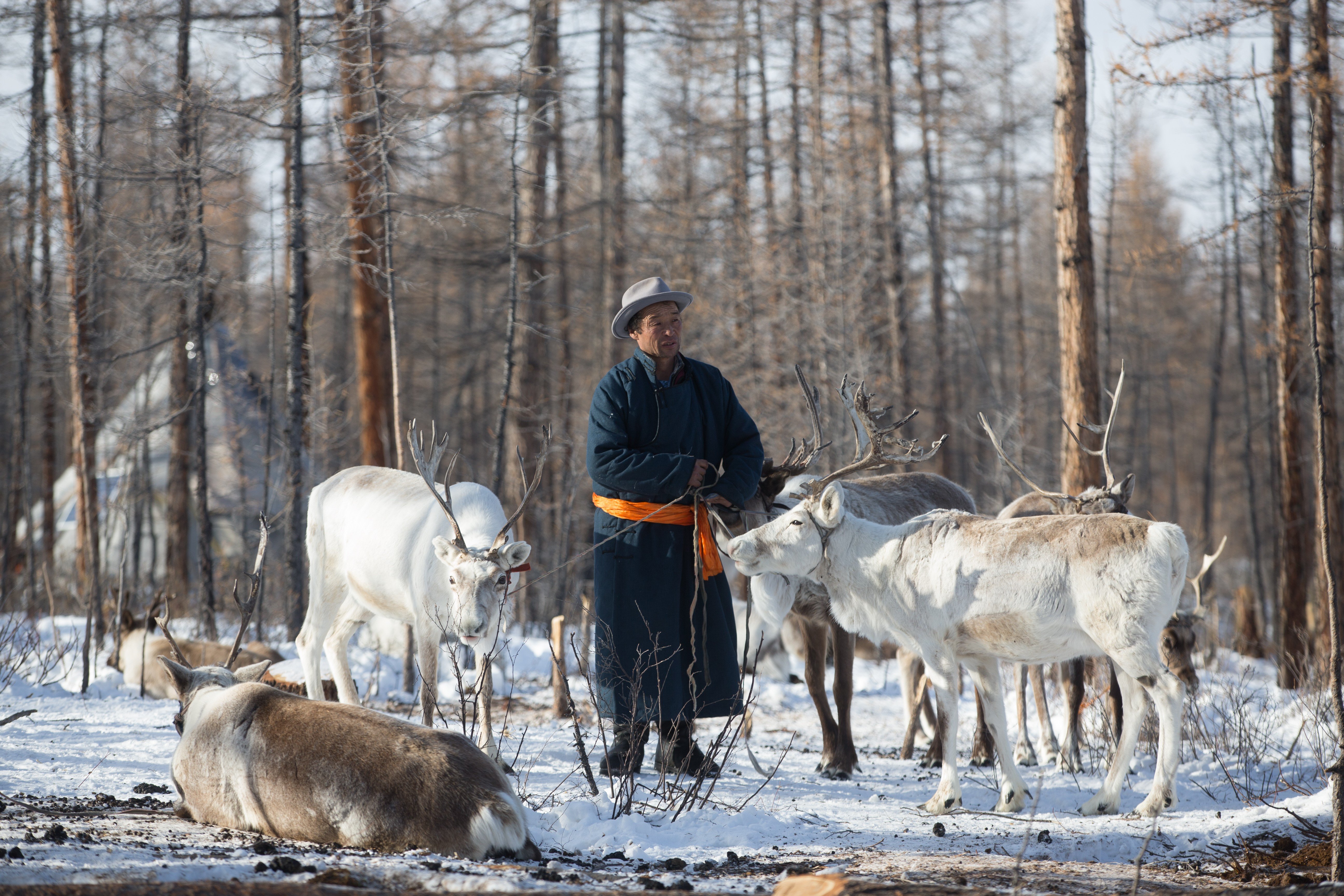This color photograph captures a detailed scene of an Asian man, dressed in a long, dark blue coat with a yellow sash, standing in the middle of a snowy forest. The trees behind him are bare, devoid of any leaves, emphasizing the wintry setting. He is wearing wool boots or moccasins on his feet and a gray fedora or similar hat on his head. The man appears to be harnessing a team of reindeer, with cords around their necks, possibly preparing to attach them to a sleigh. Among the reindeer, some are brown and others are white, with five or six standing near him and more resting in the background. The animals, with their prominent antlers, are positioned in a way that suggests they are being guided or arranged by the man.